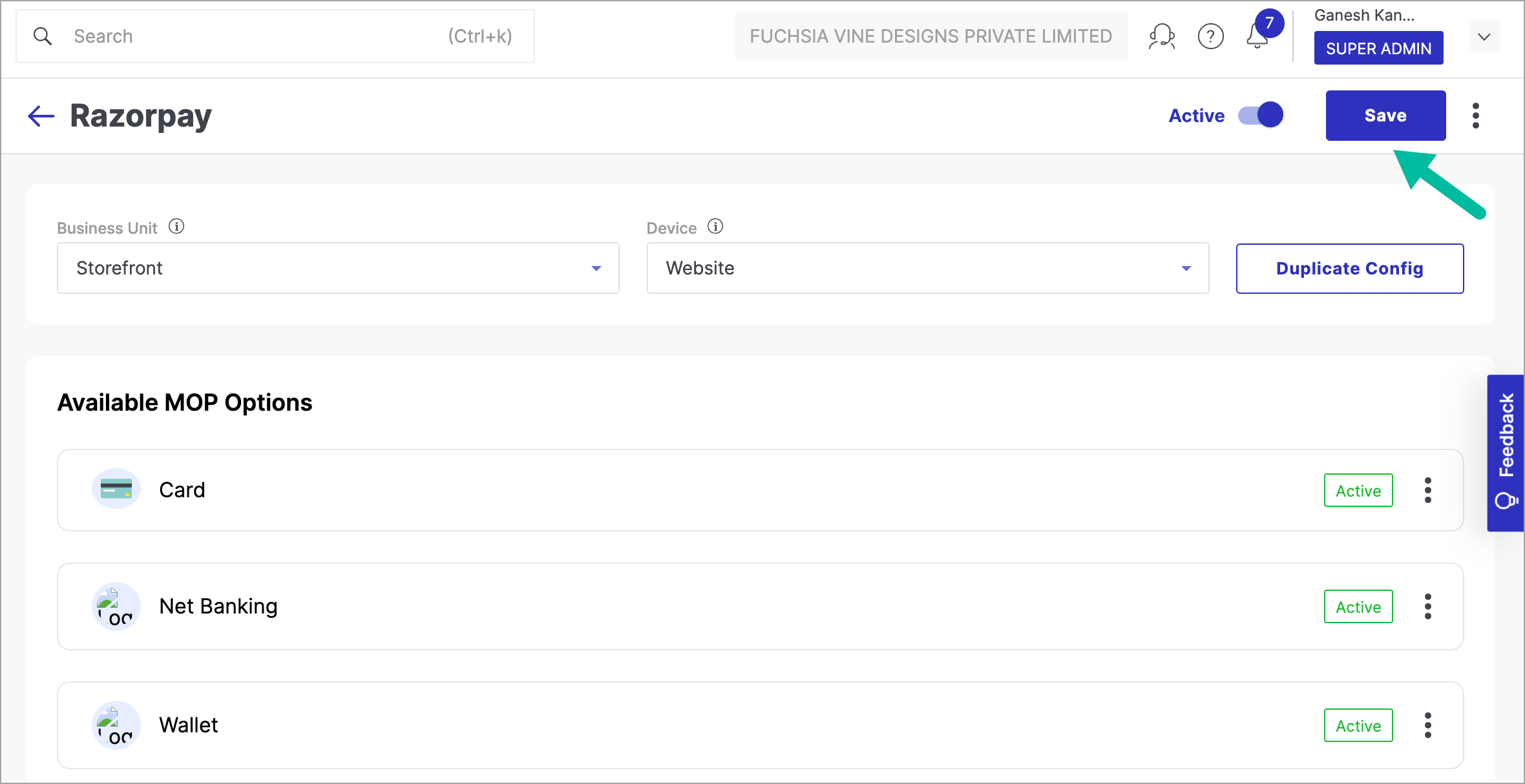This is a detailed screenshot likely from a web-based business management platform. At the top left corner, you see a search bar adorned with a magnifying glass icon on the left and the shortcut "Control + K" displayed to the right. The header contains the text "Fuchsia Vine Designs, Private Limited," accompanied by an icon of a person, an icon of a circle encapsulating a question mark, and a bell icon featuring a blue circle with a white number 7. Next to these icons, the name "Ganesh, K-A-N" appears, although the rest of the name is truncated. The title "Super Admin" is clearly visible beneath this.

Below the header, an arrow icon directs to the left adjacent to the term "Razorpay," spelled out as R-A-Z-O-R-P-A-Y, with a status indicator labeled "Active." The active status is confirmed by a slider button set to the 'on' position. A prominent blue rectangle labeled "Save" in white letters is present, highlighted with an added green arrow pointing towards it.

Further down, several sections are labeled, including "Business Unit," "Storefront," "Device," "Website," "Duplicate," and "Config." The "Available MOP options" section follows, listing payment options: "Card" (marked Active), "Net Banking" (marked Active), and "Wallet" (marked Active).

On the right side of the image, a vertically oriented blue rectangle features an icon of a light bulb, accompanied by the word "Feedback" in white letters.

There are no individuals depicted in this screenshot, emphasizing the layout and details of the interface elements alone.